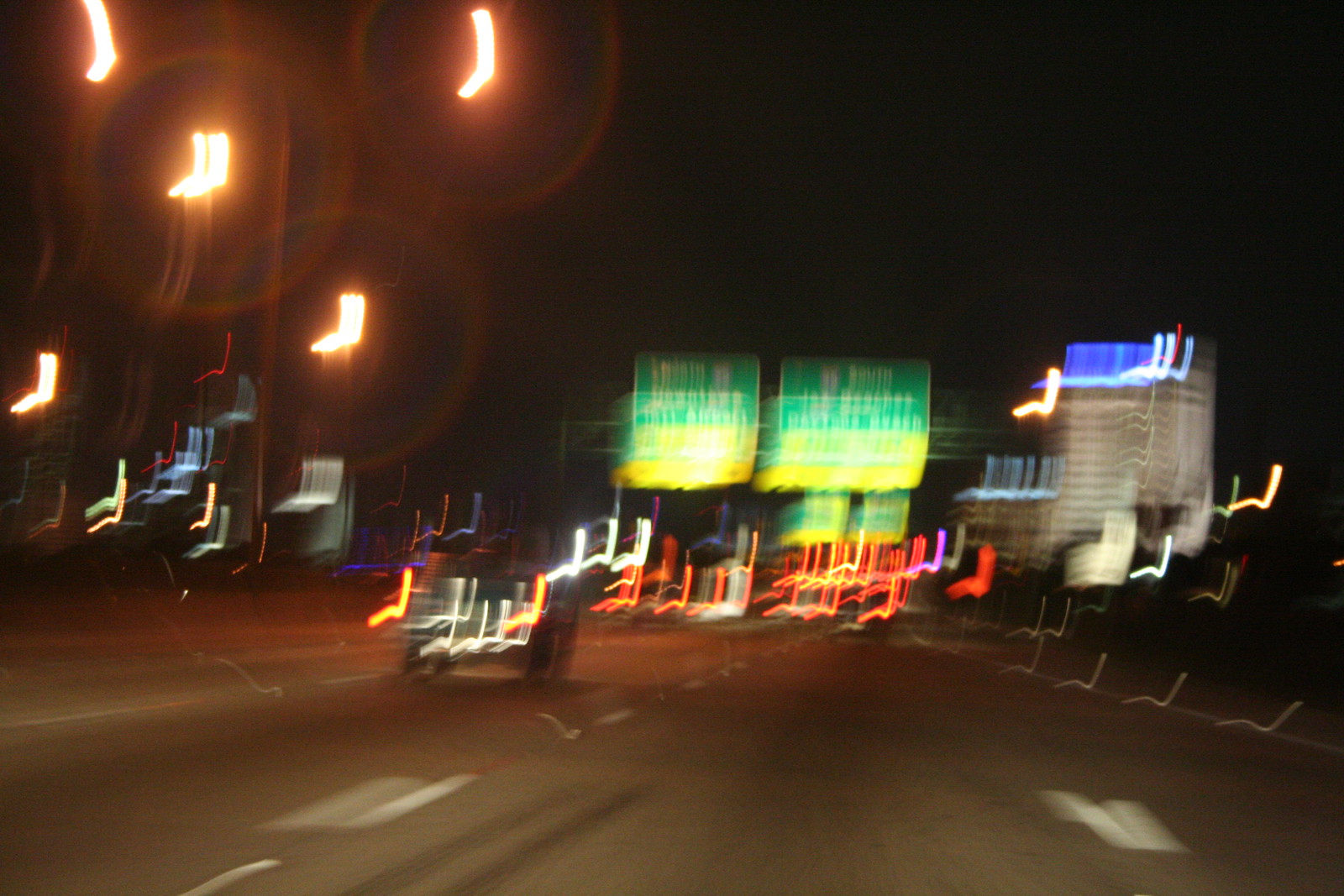This is a blurred photograph of a nighttime highway scene, seemingly captured with a moving camera that caused light trails. The sky is pitch black, highlighting the various light streaks in the image. To the left side, orange-yellow lights from highway lamps cast a glow, whereas the upper left features prominent green and yellow highway signs with white text, likely indicating exits and directions such as Interstate 35, with potential north and south routes. These signs, characterized by their green backgrounds and yellow exit indicators, add color to the otherwise dark scene. Multiple car brake lights create backward L-shaped light trails in red, white, yellow, and even some purple and blue. A large, multi-story gray building with blue lighting on its top can be seen on the right side of the image. The road below is depicted with blacktop and dashed white lane markings, guiding the blurred traffic flow ahead. The majority of the vibrant light colors and lit-up signage dominate the middle and upper parts of the scene, demonstrating a busily lit highway environment amidst the night backdrop.